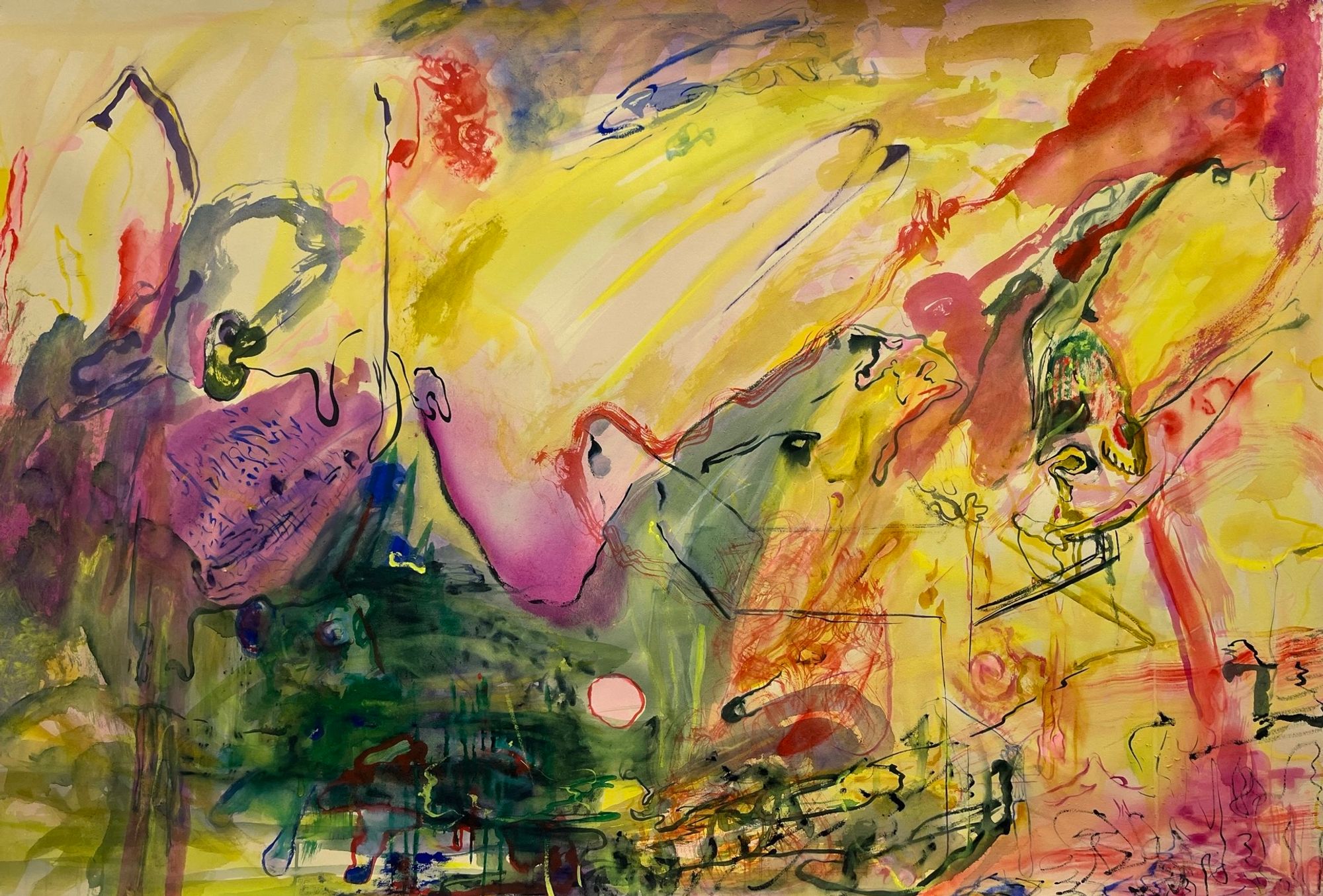This image captures a vibrant abstract painting that masterfully combines various mediums. Predominantly executed in watercolor, the artwork features a rich yellow background that sets a bright and dynamic tone. Contrasting boldly against this sunny canvas, fiery red blobs burst with intensity from several corners, infusing the piece with energy and movement. The organic shapes, outlined meticulously in black pen, add definition and structure to the fluid composition. Additionally, intricate details in pen and ink provide layers of texture and depth, while a large patch of verdant green anchors the bottom corner, offering a lush counterpoint to the dominant yellows and reds. Pencil sketches interspersed throughout bring a subtle, delicate touch to the piece, completing this complex and captivating visual experience.